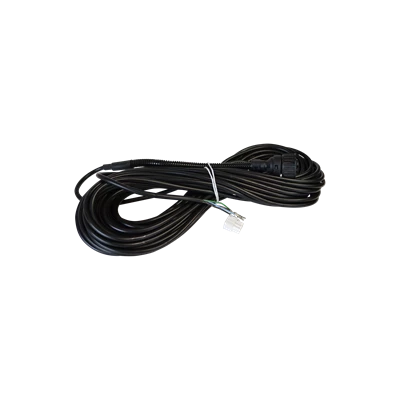The image showcases a high-tech black cable, resembling a category 6 Ethernet or possibly a phone cable, tightly coiled in a figure-eight or infinity shape against a stark white background. The cable, which appears to be about a hundred feet long, features a durable vinyl coating. It is secured at the center by a white twist tie. At one end of the cable, there's a plastic clip, clear or silver in color, suggestive of a phone jack or Ethernet plug. The opposite end hosts a larger, round black connector with ridges, potentially for twisting and securing into a device. This detailed setup hints at the cable's likely use in a commercial or high-tech application.